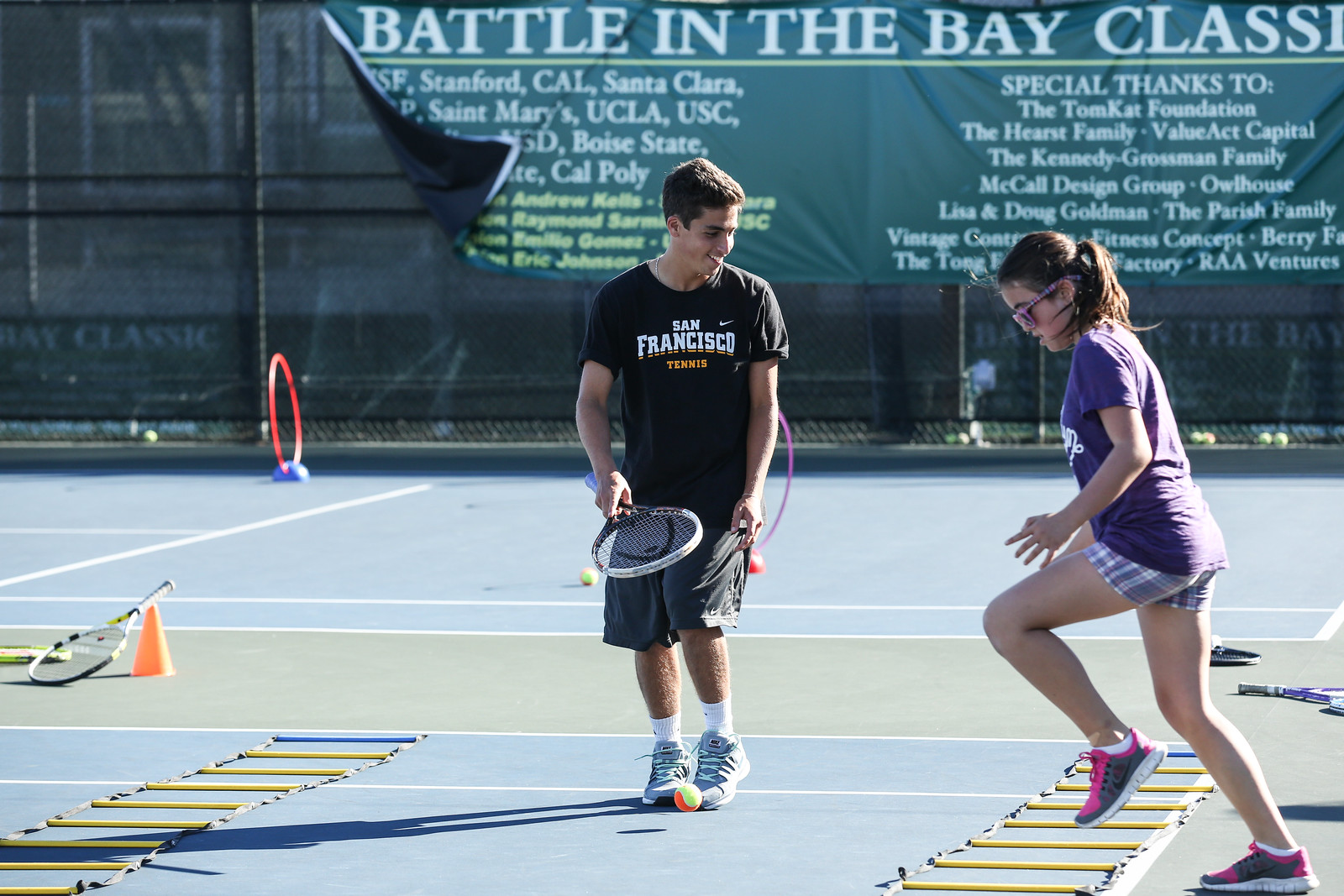In the image, two young people are on a tennis court engaging in drills. The boy on the left, dressed in a black shirt with "San Francisco Tennis" written in white, gray pants, and white shoes, is holding a tennis racket, seemingly bouncing the ball. The girl on the right, clad in a purple shirt, patterned striped shorts, and pink and gray shoes, appears to be doing exercises on a yellow rope ladder laid out on the court. A cone and various other training equipment are scattered around. In the background, a large green banner on the fence reads, "Battle in the Bay Classic" in white text, alongside lists of institutions and acknowledgments.